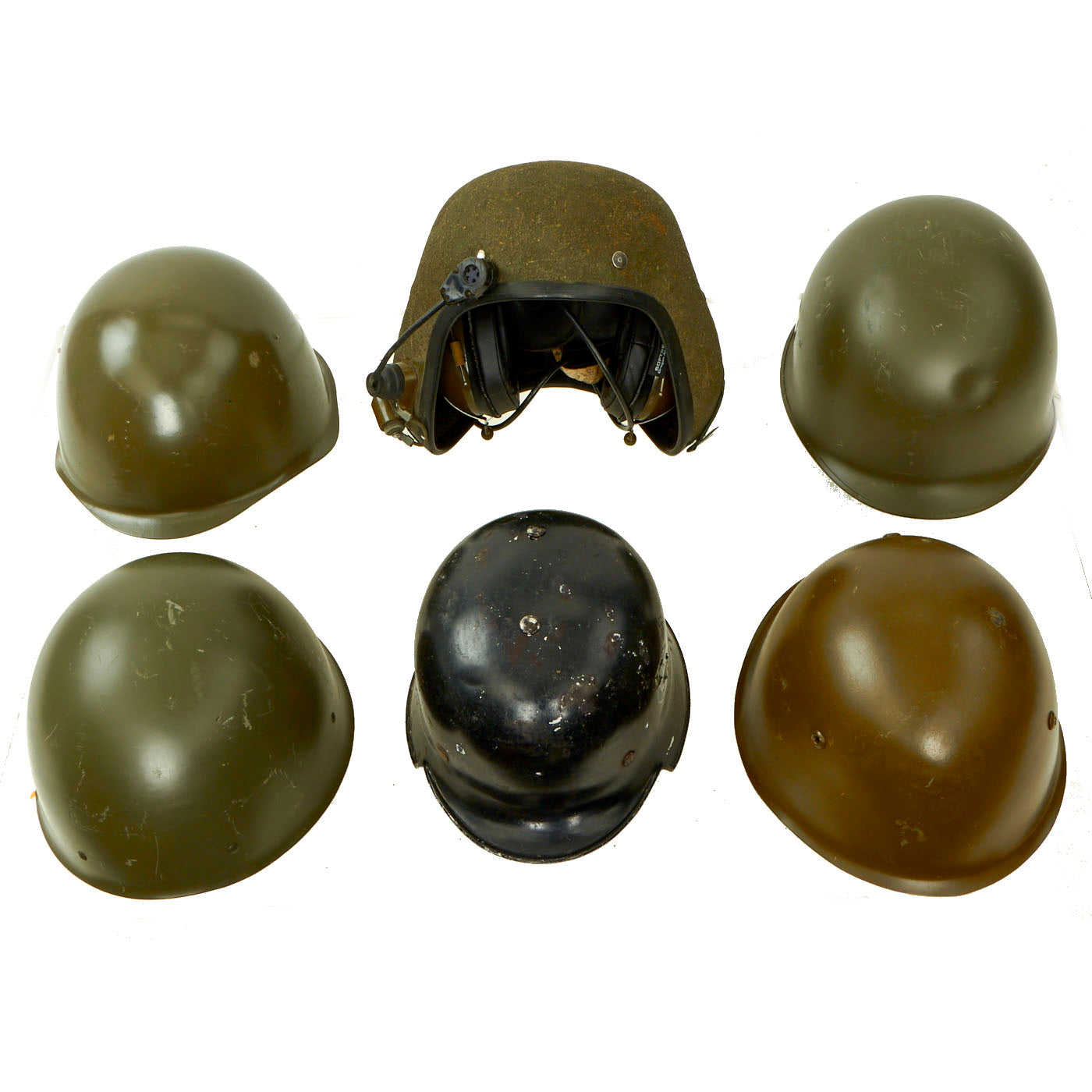This detailed photograph showcases six vintage military helmets arranged in two rows against a completely white background, presenting a stark contrast that accentuates their distinctive features. The top row includes three helmets: the one on the left is an olive-green hue, the one in the middle has a cutout for the eyes and sides that extend to cover the ears, crafted in a gold-olive green shade with black plastic areas around the eye openings and appears to be equipped with a soft composite material and potentially some old communication equipment including a wire and a microphone, while the helmet on the right is a deeper olive-green color. The bottom row also displays three helmets: the left helmet mirrors the olive-green tone of its top-row counterpart, the central helmet is black with visible rust and pitting indicative of its age, and the right helmet diverges in color with a brighter copper-like tint. All helmets, except for the center one in the top row, are placed face down, revealing only their dome-shaped tops, displaying evident signs of wear such as scratches, dents, and chipped paint. The central helmet on the top row stands out with its more complex structure and eye cutout, adding a layer of historical intrigue to this evocative assembly of military relics.